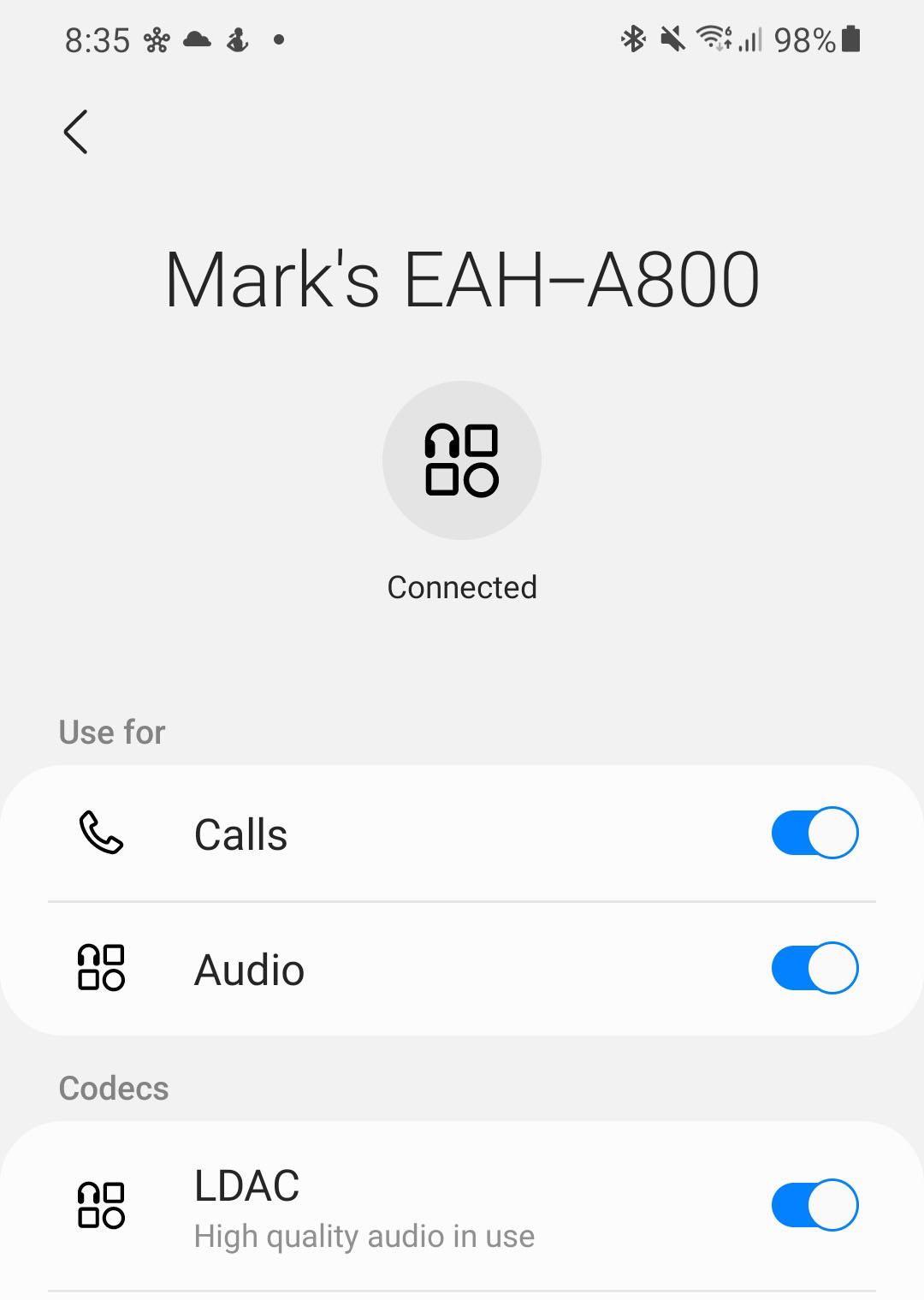This image is a detailed screenshot captured from a smartphone at 8:35 AM. The top status bar features several icons: a snowflake icon indicating a weather notification, a jogging woman icon, and a dot icon. Towards the right side of the status bar, additional icons include Bluetooth, a muted phone icon, Wi-Fi, and a possible roaming or Wi-Fi calling icon, with the phone showing a signal strength of three out of four bars. The battery icon displays a 90% charge. The text "Marks EAH-A800 connected" suggests that a Bluetooth device named Marks EAH-A800 is currently connected to the phone. Detailed information for this device includes options for calls, audio, and LDAC codecs with high-quality audio selected. The background of the image is predominantly white. The section for the Marks EAH-A800 displays a 2x2 grid of icons. The top left icon depicts headphones in a square, while the icon below it shows a circle within a square, indicating various audio and LDAC settings.